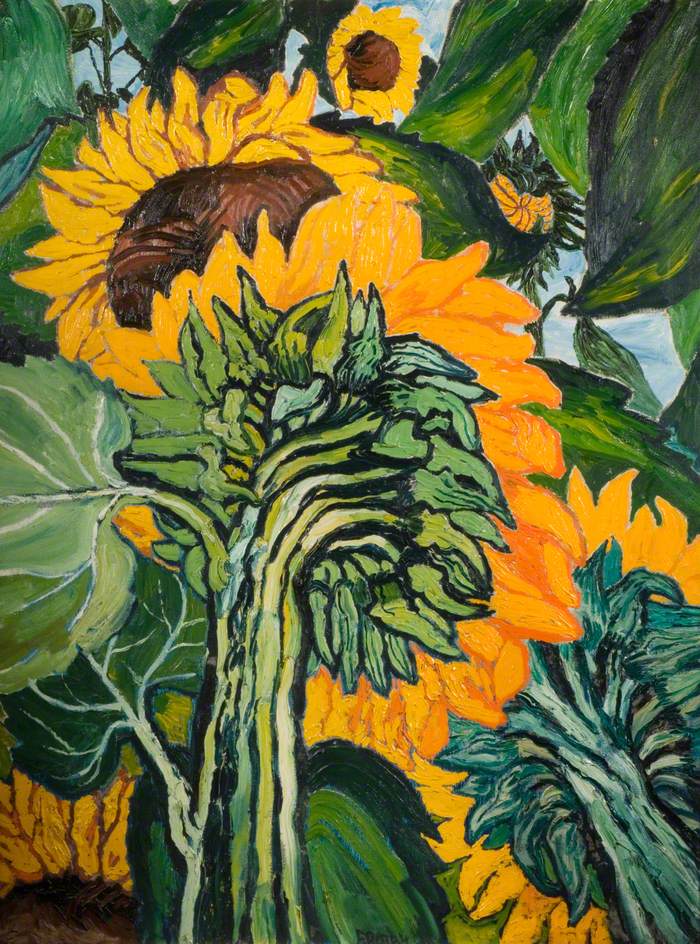This impressionistic artwork depicts a vibrant sunflower garden, likely in the style of Van Gogh. The painting prominently features three or four large sunflowers with bright orangish-yellow petals and rich brown centers. These sunflowers are surrounded by dynamic green foliage, accented with bold black lines, enhancing their visibility. The composition includes both front-facing sunflowers and several viewed from the backside, capturing different perspectives. Smaller flowers and detailed leaves also appear in the foreground. The background showcases a blue sky with scattered puffy white clouds, suggesting a pleasant day. The overall effect is a vivid, close-up portrayal that may be a detail from a larger piece, emphasizing the beauty and texture of the sunflowers against a serene sky.